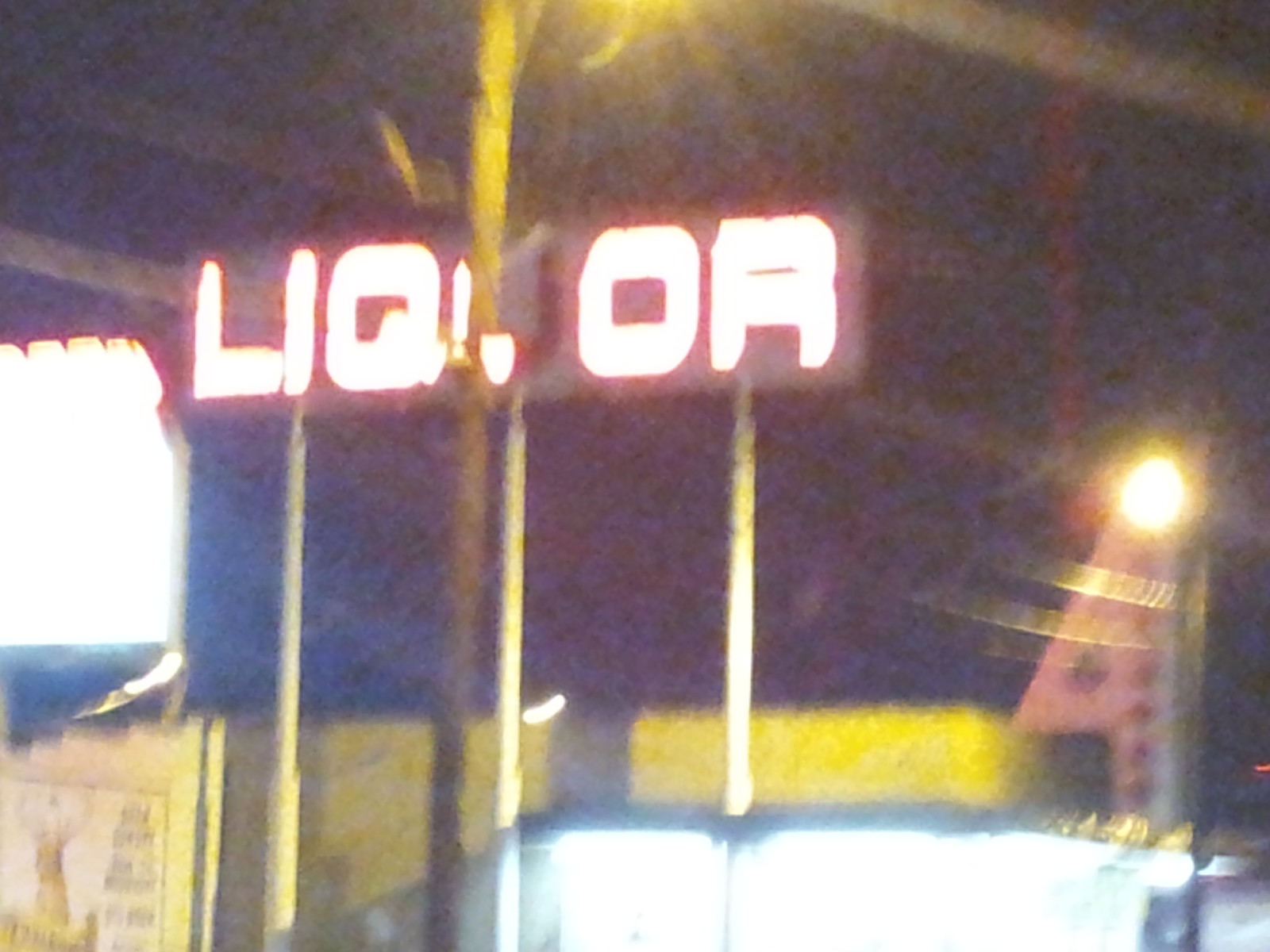The photograph is a blurry, nighttime image taken outside a liquor store with poor focus and a hazy background. The main feature is a brightly lit neon sign with the word "LIQUOR" in reddish neon lettering, though half of the letter "U" is obscured, possibly by a power line or tree trunk. This sign is supported by three metal poles, which some descriptions suggest are yellowish. The bottom right corner might show the actual store, which is also very brightly lit but unclear due to the blur. Beside the liquor sign, to the left, there is another too-bright-to-read LCD screen adding to the glare. Multiple street lamps are visible, contributing to the overall glare in the scene. Power lines are also barely visible at the top of the image, and the sky is dark, indicating that the photo was taken late at night. There are indistinguishable yellow square-like objects and other frame-like structures at the bottom, which are not clearly identified. The low quality and possible motion blur of the image suggest it was taken either through a window or with a low-grade camera.